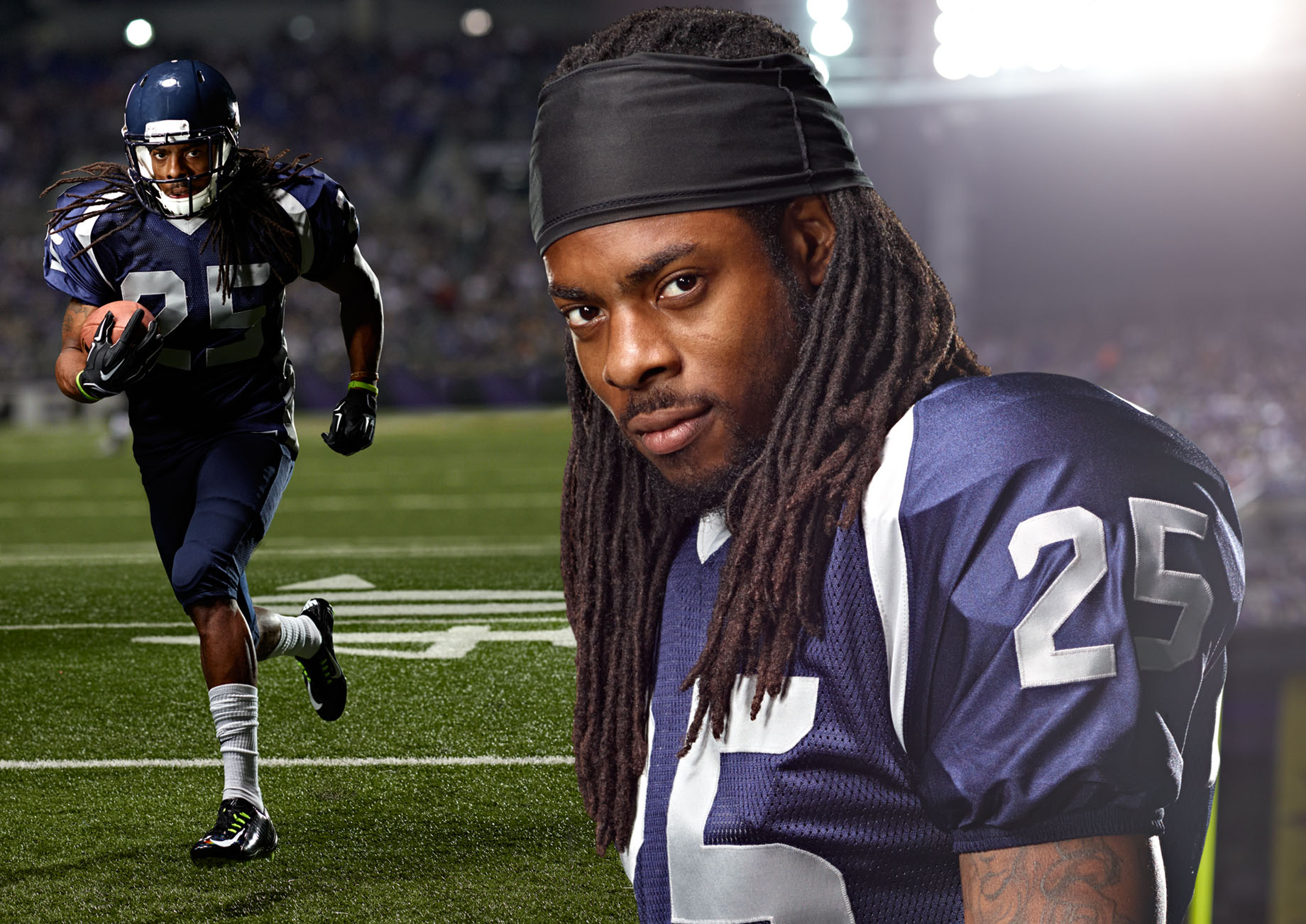The image showcases two pictures of NFL player Richard Sherman from the Seattle Seahawks, depicted in distinct moments on the football field. On the left, Sherman is captured in mid-action running with a football, dressed in a navy blue uniform complete with helmet, gloves, and cleats, and the number 25 visibly emblazoned on his chest. The background reveals the number 40 painted on the AstroTurf Green field. In contrast, the right side of the image zooms in on Sherman's face, presenting him helmetless with a slight smile, wearing a black bandana and revealing a tattoo on his arm. His black dreads cascade around his shoulders, highlighting his focused yet relaxed demeanor. The uniformity in his attire across both images emphasizes the team's blue and lime green color scheme, juxtaposed with the green, white, brown, and black of the football field.